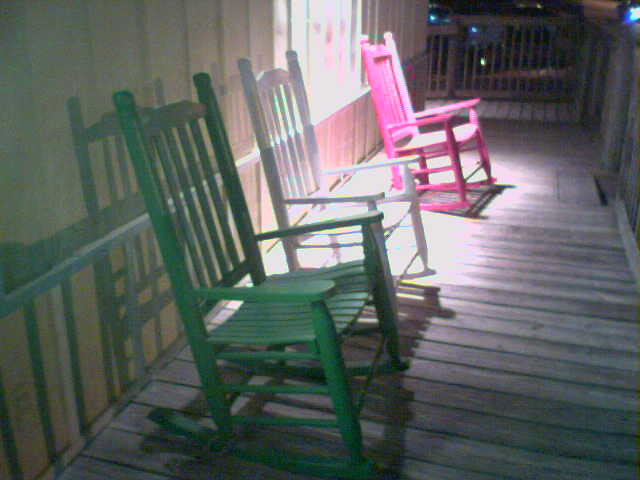The image depicts a nighttime scene of a wooden patio deck, likely part of a restaurant, illuminated by a light shining down from above. On this deck are three distinct rocking chairs, painted green, white, and pink, respectively. The green rocking chair closest to the photographer, followed by the white one, and then the pink one at the far end. The chairs are positioned against a tan-colored wood wall or siding with white trim, casting shadows that suggest a brown hue. The deck features visible wooden planks and is enclosed by a wood fence. In the background, a parking lot with one parked car is noticeable, and there are multiple blue lights emanating from the top right of the image. Between the pink and white rocking chairs, a window reflects some of the ambient light, adding to the scene's cozy yet slightly blurry ambiance.